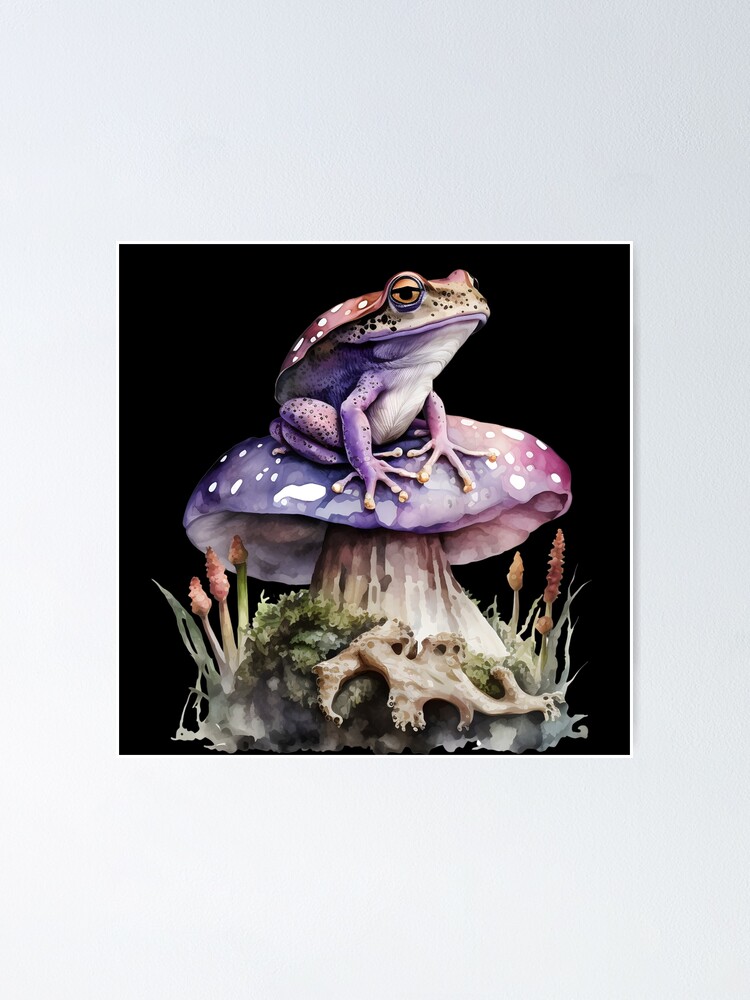In the detailed imagery, we see a vibrant frog perched atop a substantial Amanita mushroom, possibly rendered through digital art or hand painting. The amphibia exudes a unique gradient hue, transitioning from purple on its underside to a greenish tone towards its top, culminating in a burgundy-red back adorned with white polka dots. This coloration mirrors the mushroom it rests upon. The frog’s face is beige with black specks, highlighted by black-rimmed eyes with black pupils and yellow-gold sclera.

The Amanita mushroom is prominent in the composition, about twice the size of the frog. It displays a captivating color palette, merging purples and reds with white spots sprinkled across the cap. The thick, yet short stem reflects a gradient of beiges and browns. The mushroom grows out of lush green moss, surrounded by an array of terrestrial details including potential mycelium growth or artistically depicted sticks.

The surrounding environment adds to the detailed setting with blades of green grass on either side of the mushroom and small plants featuring red bulbous tips. There are also delicate flowers with green stems, showcasing varying shades of pink to pale peach, reminiscent of hyacinths or bluebonnets. The backdrop includes a stark color contrast—a predominantly white background with a central black section anchoring the vivid colors of the frog and mushroom, creating a striking and intricate visual display.